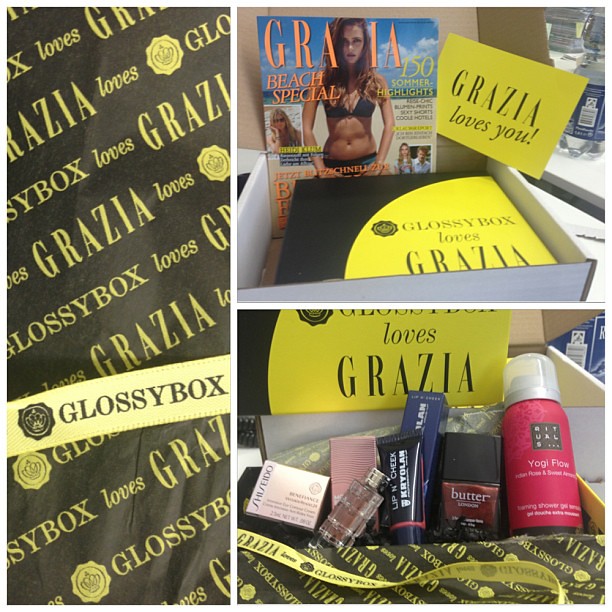This image is a detailed collage featuring three distinct sections, focusing on a beauty subscription gift set collaboration between Grazia and Glossy Box. 

On the left side of the image, a black background is adorned with yellow, diagonal text repeatedly declaring "Grazia Loves Glossy Box", interspersed with a thin black ribbon stating "Glossy Box" in white letters.

The top right section showcases an open white subscription box. Inside, a prominently placed magazine cover features a bikini-clad woman under the headline "Grazia Beach Special," with the background text "Grazia Loves You" written in the same yellow and black motif. A small card inside also reads "Glossy Box Loves Grazia."

The bottom right portion details the contents of the subscription box, displaying seven different beauty products. Among them are items such as Shiseido, a small perfume bottle, a product labelled Kyrolam, nail polish from Butter, and a pink-bottled item named Yogi Flow. The arrangement highlights the variety and high-end nature of the included products.